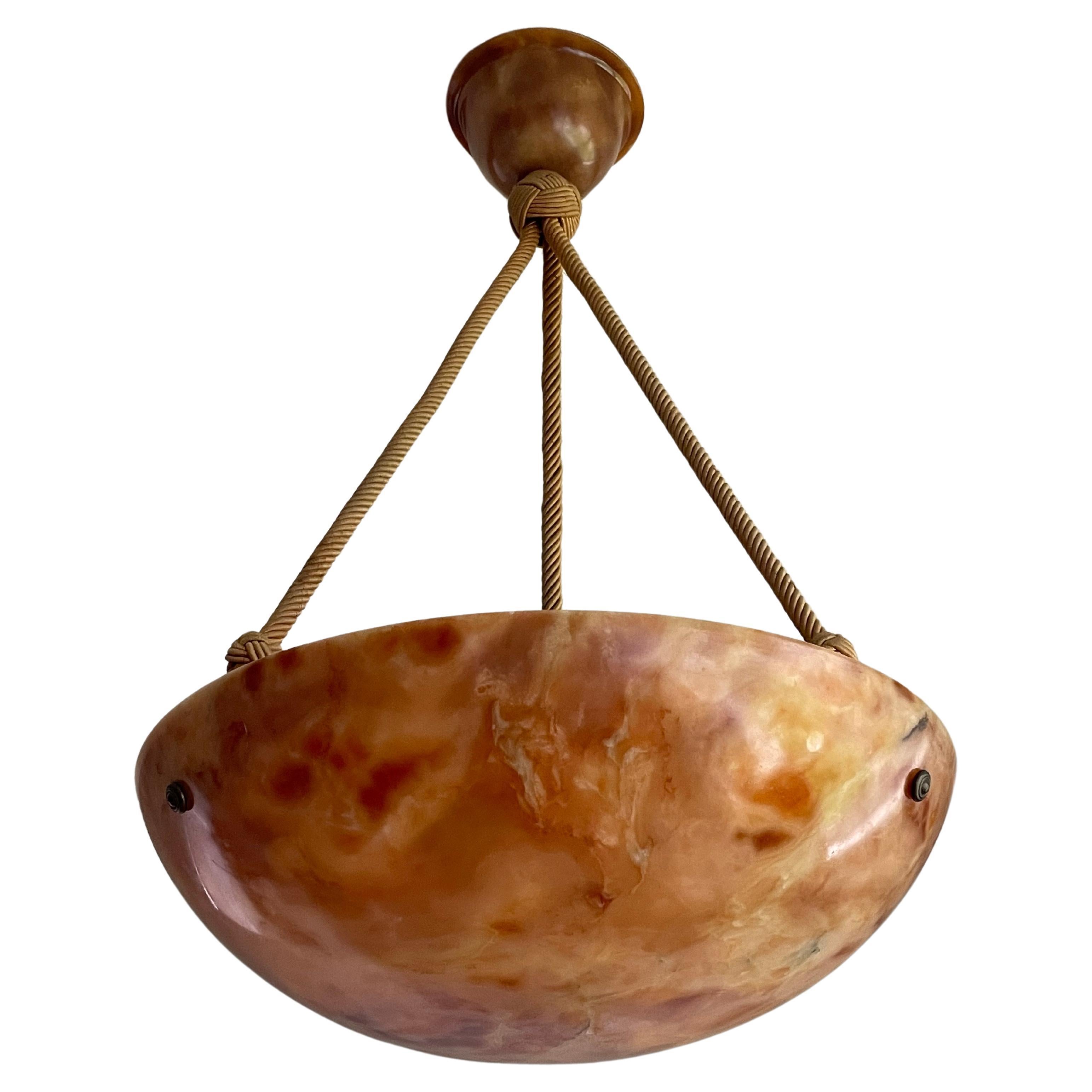The image captures a modern chandelier with a distinct marble-like appearance, hanging from the ceiling. The fixture has an opaque dome shape, resembling a large bowl with swirls of yellows, oranges, peaches, and rust colors. The chandelier is suspended by three matte gold ropes, which appear twisted and sturdy, converging at a brass-like ceiling fixture that resembles an upside-down bell. The image is taken from an underneath perspective, giving a clear view of the intricate patterning on the chandelier. The background is whited out, lending an edited appearance to the photo, and just beside the light fixture, there's a peculiar formation resembling a small alien face.